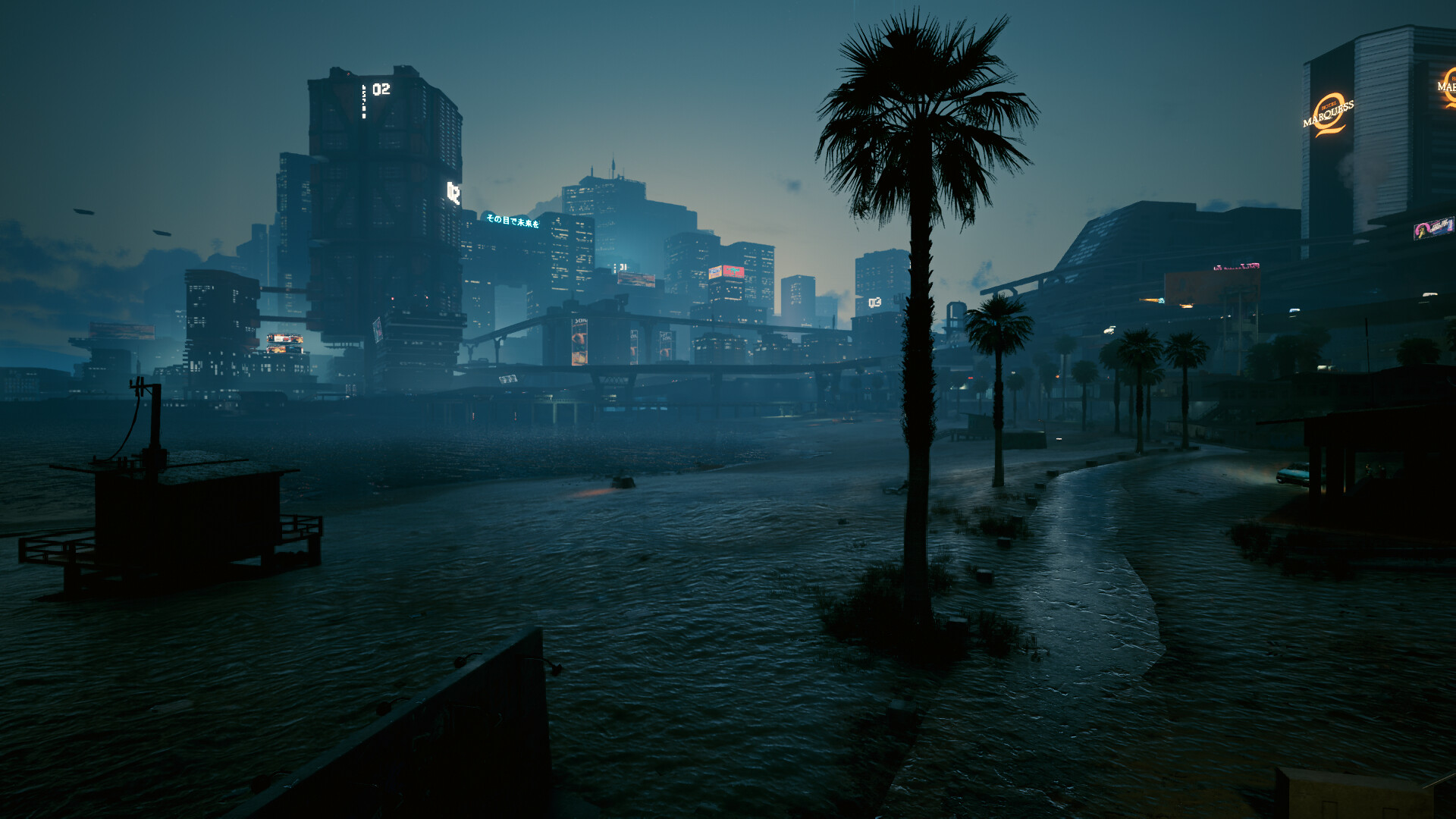This image features a striking, blue-toned scene reminiscent of the Grand Theft Auto (GTA) game series, specifically evoking the vibe of a beach setting within the game. Dominating the background are several tall palm trees, swaying gently and adding a tropical atmosphere. Various buildings can be seen, each adorned with signage that enhances the urban beach ambiance. A single car is visible with one headlight flashing, while the other is off, which further suggests a virtual, possibly in-game environment. The overall composition and the distinct color grading contribute to the impression that this is a meticulously crafted scene from a video game, rather than a photograph from real life. Regardless of its origin, the image captivates with its tranquil yet vibrant beauty, making it an appealing choice for a screensaver.